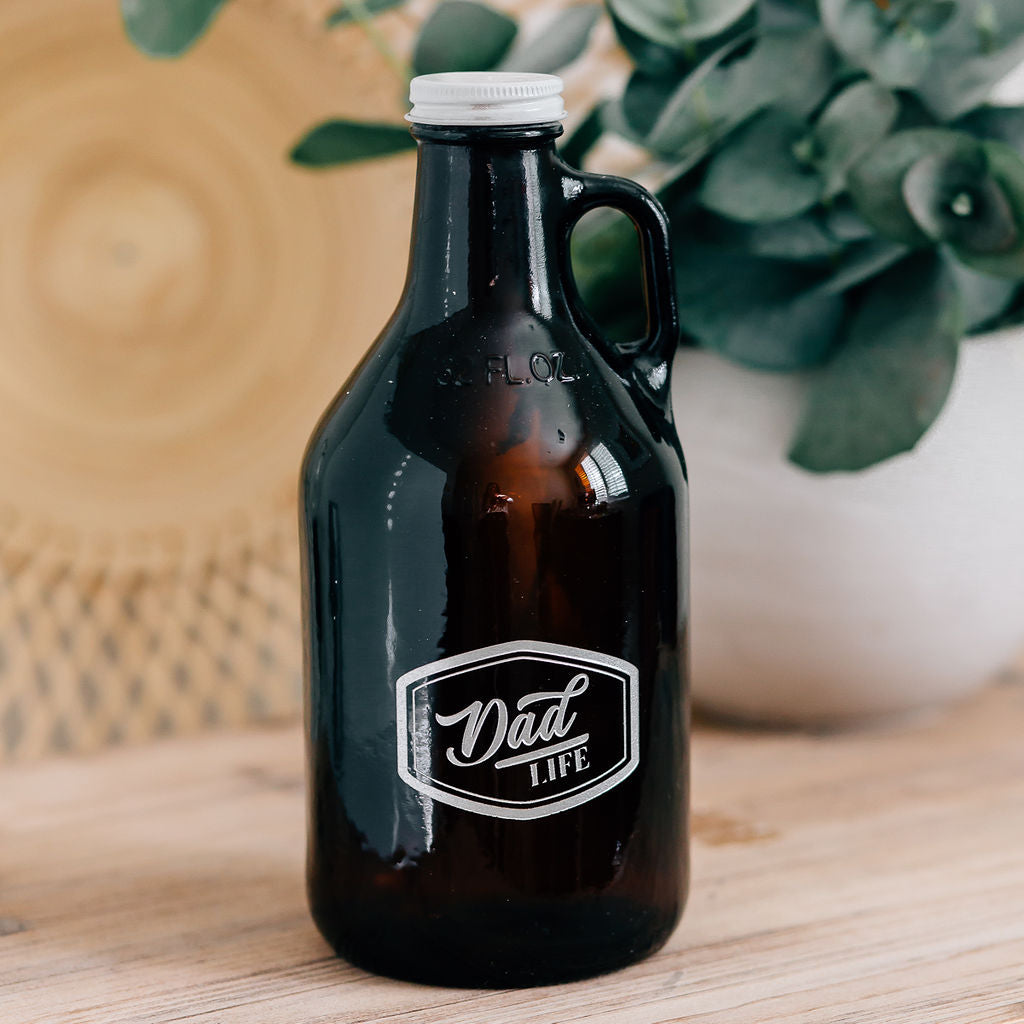This detailed indoor photographic image prominently features a distinctive brown glass jug bottle with a white screw cap, which is likely metal and appears to secure with a single turn. The bottle, somewhat stubby and stout, includes a small handle extending from the neck to its wider body. The center of the bottle proudly bears a hexagonal emblem with the text "Dad Life" written in white. Above this emblem, near the neck, the bottle indicates its capacity in fluid ounces, assumed to be around 20, although the exact number is slightly obscured. The bottle sits on a light brown wooden table. The background is artistically out of focus, featuring a white planter with lush green plants and, to the left, part of a wicker chair. The bottle also reflects a window from the surrounding room, drawing attention to its smooth, polished surface.